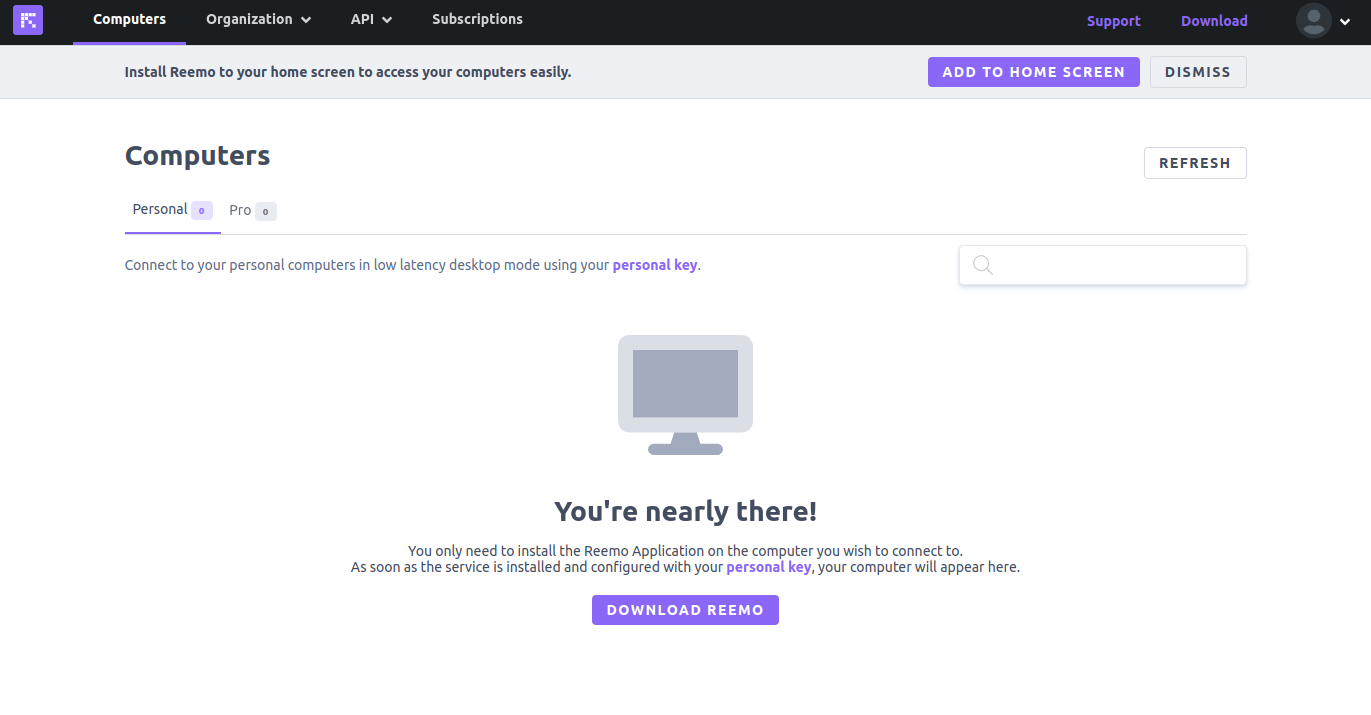**Detailed Descriptive Caption:**

The image is a color screenshot, likely from a website or computer settings interface. At the very top, there's a black band featuring a square icon with a pixelated arrow pointing to the top-right corner. The arrow is white, set against a purplish square background. Next to this icon is some white text, alongside a tab with a highlighted purple underline indicating the current selection. The tab options include "Organisation," "API," and "Subscriptions." 

On the right side, the header contains options such as "Support" and "Download," both in purple text. Additionally, there’s a circular user icon displaying a head-and-shoulder silhouette, accompanied by a down arrow for user profile options.

Below this, the main section consists mostly of black text on a white background. A prominent message at the top reads, "Install remote to your home screen to access your computers easily." To the right of this message are two buttons: a purple one labeled "Add to home screen" in white text, and a white one labeled "Dismiss" in black text.

Following this section, on the left, the word "Computers" is present, with a "Refresh" option on the right side. Beneath these, "Personal" and "Pro" categories are displayed, with "Personal" being selected, indicated by a blue or purple underline. The text under "Personal" states, "Connect to your personal computers in low latency desktop mode using your personal key." The term "personal key" is highlighted in purple.

Adjacent to this, there is a greyed-out search box on the right. Below this main section, an icon resembling a computer screen is centrally positioned. Within this icon, the text reads, "You're nearly there. You only need to install the remote application on the computer you wish to connect to." It further explains that once the service is installed and configured with the "personal key" (highlighted in purple), the relevant computers will appear in this section.

Finally, at the bottom center of the image, there is a prominent purple button with the white text "Download remote."